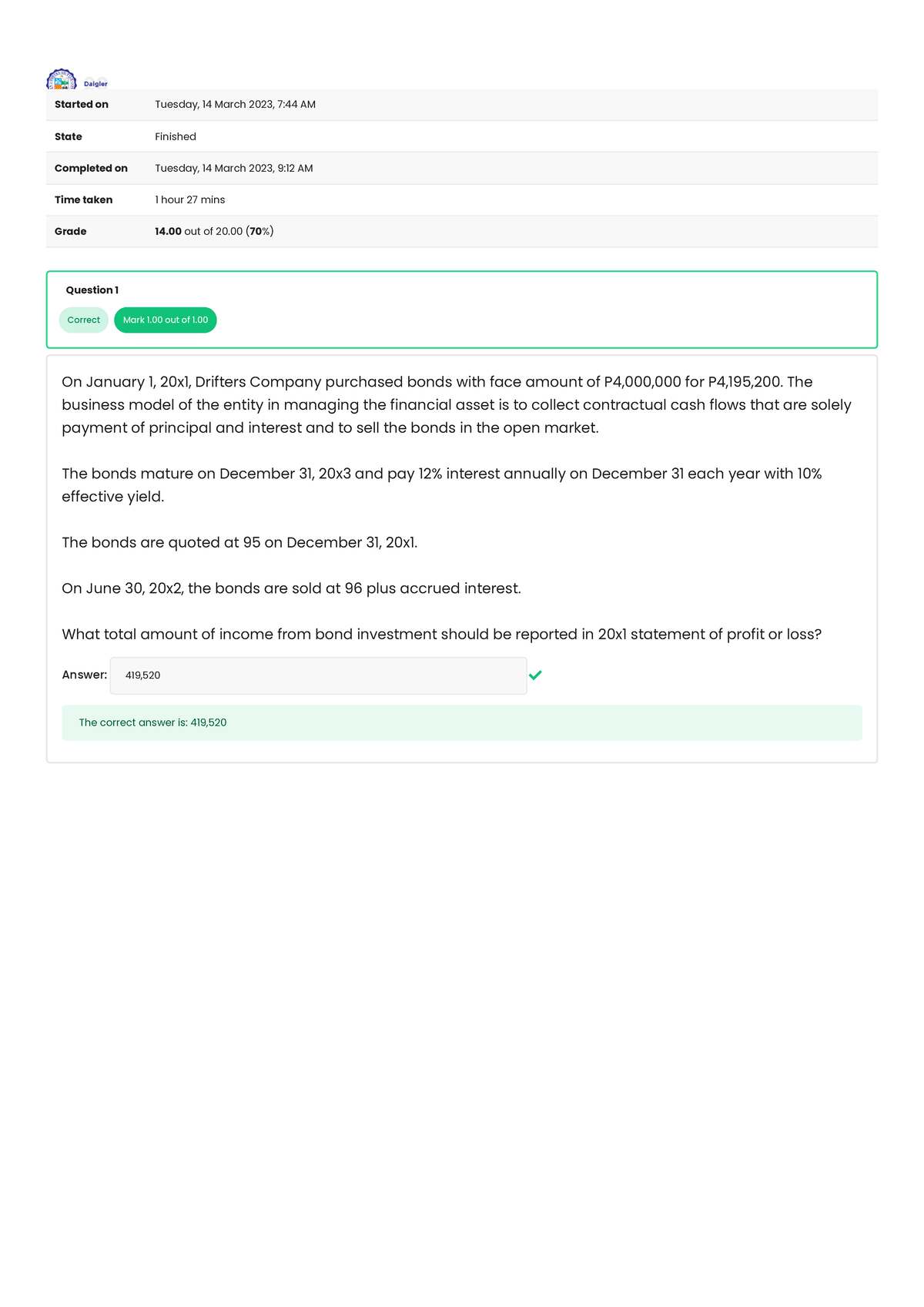This detailed and descriptive caption relates to the screenshot of an examination result from Daigler, which appears to be associated with a university or college. 

---

**Screenshot Caption:**

The screenshot displays an examination result from Daigler, identifiable from the crest and the name located in the upper left-hand corner. The content of the screenshot includes detailed information, subdivided into various sections marked by alternating gray and white rows. All topical headings are in bold, with corresponding entries in regular black font.

1. **Started:** Tuesday, 14 March, 2023, 7:44 AM
2. **State:** Finished
3. **Completed On:** Tuesday, 14 March, 2023, 9:12 AM
4. **Time Taken:** 1 hour 27 minutes
5. **Grade:** 14 out of 20 (70%) - both values are bolded.

Below these details, the examination questions and their corresponding responses are presented within outlined boxes.

### Question 1:
- **Question Description:** 
  - The box outlines a detailed financial problem involving Drifter's Company's bond purchase on January 1st, 20x1, with specified numbers for face amount, interest rates, maturity date, and selling conditions.
  - The question asks for the total amount of income from bond investment to be recorded in the 20x1 statement of profit or loss.

- **Answer:**
  - **Provided Answer:** 419,520 (displayed in a gray box with a green check mark to the right indicating correctness).
  - **Correct Answer Confirmation:** The answer is reiterated in a light green box with dark green text stating: "The correct answer is: 419,520."

---

This structured breakdown captures the pertinent details visually presented in the original screenshot for a comprehensive understanding.